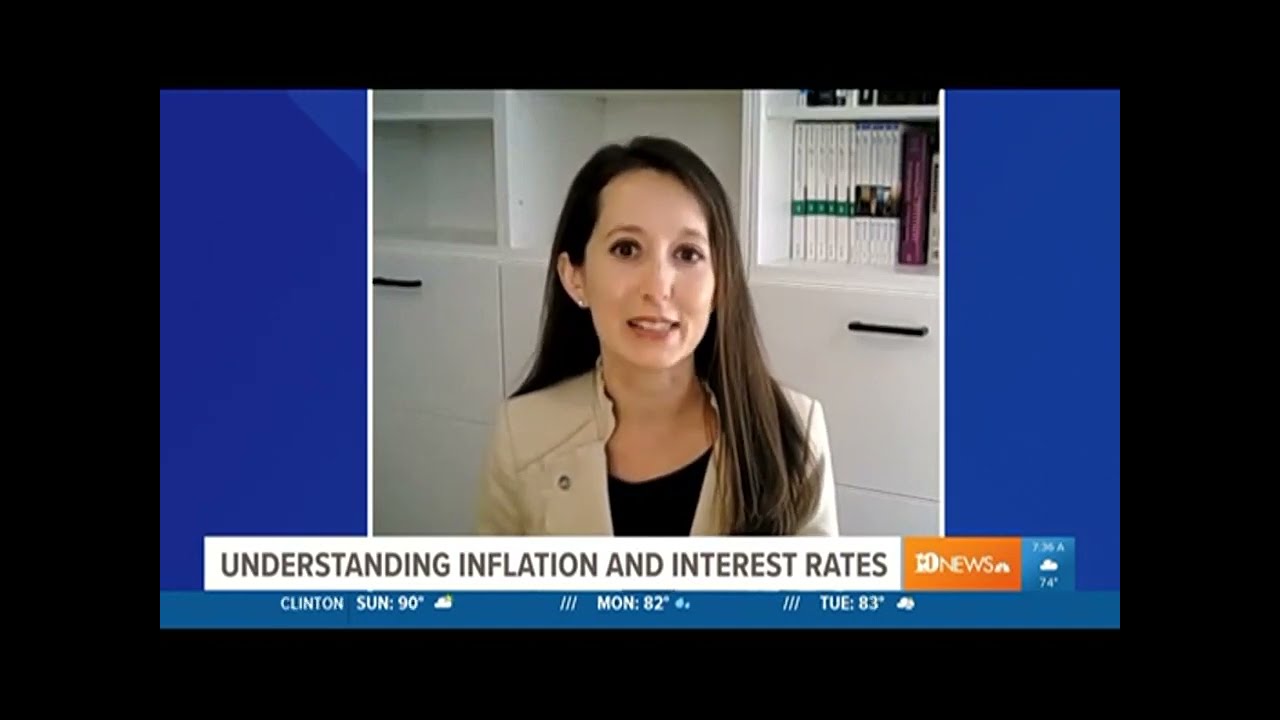The image is a screenshot of a news broadcast from Channel 10 News, featuring logos from MSNBC. In the center of the frame, a square image shows a well-groomed woman with long, straight brown hair, wearing a beige jacket over a black t-shirt. She is speaking directly to the camera against a backdrop of a white bookcase. The background surrounding her image is a bright, royal blue color. Below her photo, a white banner with black text states, "Understanding Inflation and Interest Rates." To the right of the banner, there's a weather icon showing a temperature of 74 degrees with an adjacent weather summary displaying "Clinton, Sun, 90 degrees," along with forecasts for Monday at 82 degrees with raindrops, and Tuesday at 83 degrees with some clouds. The setting of the broadcast is Clinton, although the state is not specified.